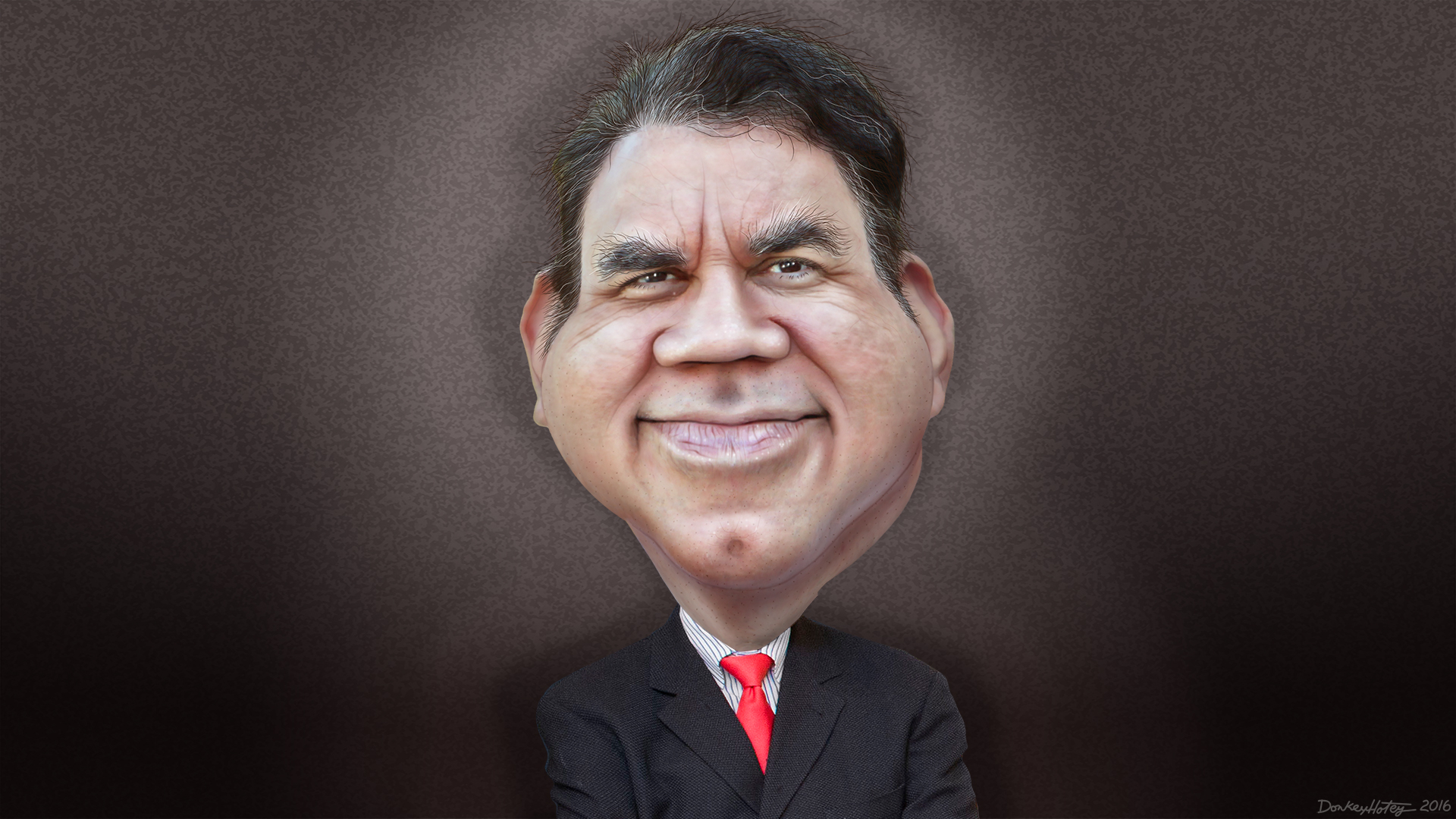In this image, there is an incredibly realistic yet cartoonish caricature of an old man who appears to be an important or familiar political figure. The exaggerated drawing features a thin, narrow body wearing a black suit with a white dress shirt and a bright red necktie. The figure's head is disproportionately large and wide, with chubby cheeks, a wide nose, and very thick eyebrows giving it a distinctive balloon-like appearance. The man has black hair and a warm, smiling expression. The background of the image is textured dark brown, contrasted by a soft, light brown halo around his head and body, creating a glowing effect. In the bottom right corner, there is an artist's watermark in white text that reads “Don Quixote 2016.”